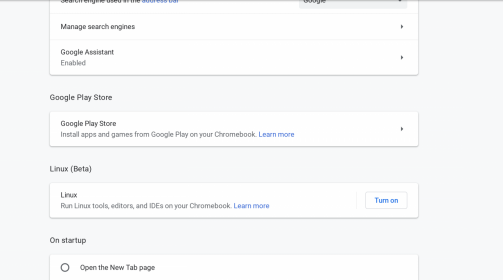The image captured appears to be a partial screenshot of a settings page from either a website or an app, featuring a predominantly light gray background. At the center of the image are various informational and interactive boxes. 

The top box is mostly cut off, but two options are visible in black text. The first option is "Manage search engines" and the second is "Google Assistant enabled."

Below this, there is a section dedicated to the Google Play Store. This section includes a rectangular box with the text "Google Play Store" inside it. Accompanying it is a brief description: "Install apps and games from Google Play on your Chromebook" followed by a blue hyperlink labeled "Learn more."

Further down, there is a text entry for "Linux (Beta)" with a corresponding description that reads, "Run Linux tools, editors, and IDEs on your Chromebook." This section also includes a blue hyperlink labeled "Learn more" and a white button with blue text that reads "Turn on."

At the bottom of the image, another section labeled "On startup" is partially visible. The only decipherable option within this section is "Open the New Tab page."